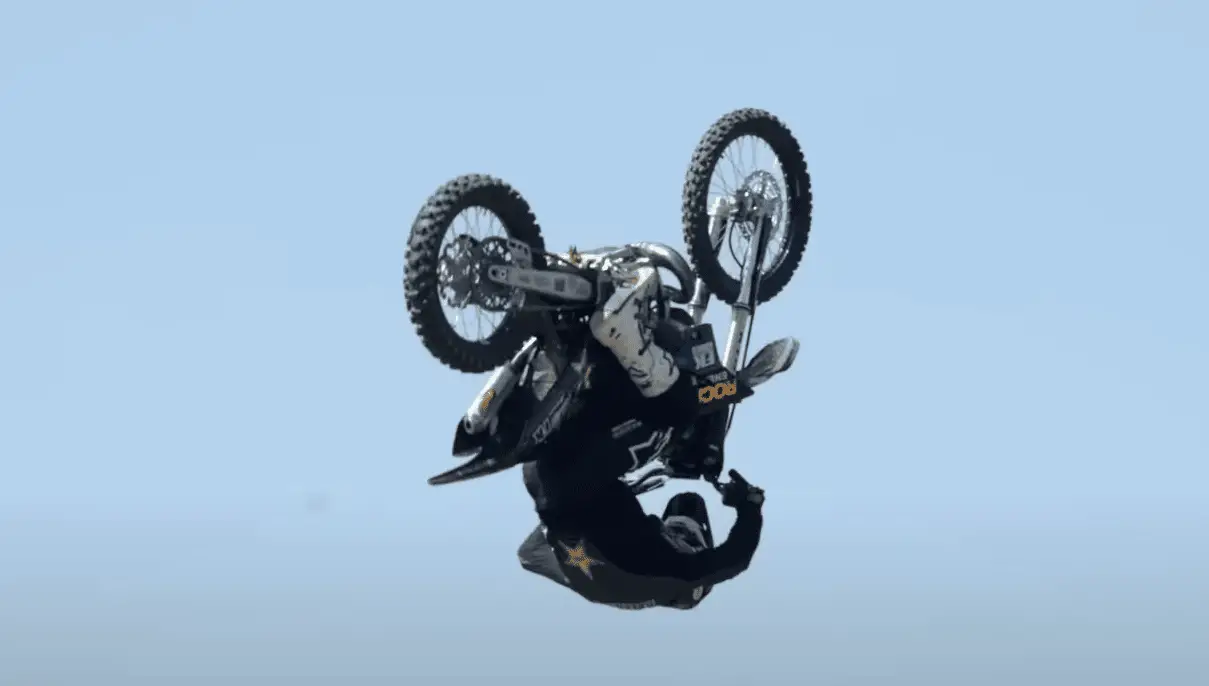Against a backdrop of a clear, light blue sky without any clouds, an action-packed photograph captures a motorcyclist mid-flip. The motorcyclist is upside down, riding a predominantly black and silver motorcycle with accents of orange. The photo's viewpoint, angling upwards, excludes any ground, ramps, or people, focusing solely on the airborne subject. The motorcycle features thin silver spokes emanating from its hubs and a motor attached to the rear wheel.

The rider, dressed in a black suit and helmet, is also inverted, showcasing a yellow star on the back of his suit. His white mid-calf boots are prominently visible, with one clearly distinguishable. Gripping the sides of the motorcycle with bent knees, the rider holds onto the upside-down handlebars. The image appears like a freeze-frame from a high-octane video, emphasizing the dynamic motion of the stunt against the serene, monochromatic sky.